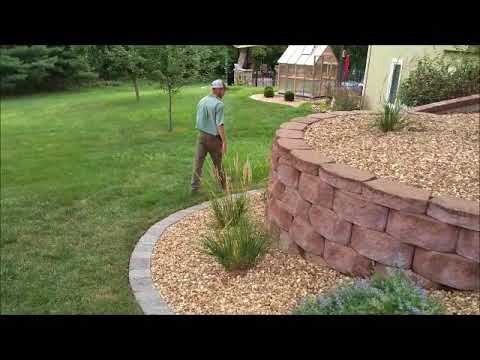In this daytime image set in a manicured backyard, a middle-aged Caucasian man, wearing khakis, a light blue long-sleeved shirt, and a white ball cap, walks away from the camera, positioned centrally. The foreground features a lush, green lawn with shrubbery and trees on the upper left-hand side. To the right, there's a stone retaining wall topped with mulch and spiky plants, enclosed by grey brick pavestones. Further back, a clear greenhouse stands in the right-hand corner. The scene is bright and vibrant, with various shades of green, brown, and additional colors like red and orange, all captured beneath a clear daytime sky. The entire setting is framed with a black border.